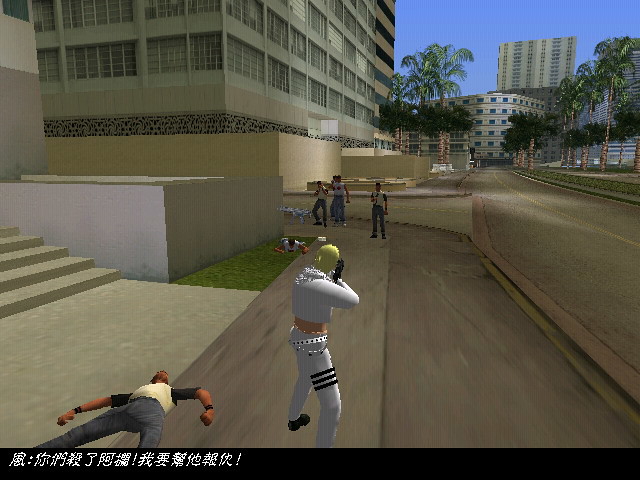In this dynamic scene from a video game, a central character with blonde hair stands poised, dressed entirely in white and holding a gun in a ready position. Lying behind them is a lifeless body, clad in gray pants, a white shirt, and dark sleeves, indicating a recent altercation. Ahead of the armed figure, four others also dressed in white are positioned; one is crouching on a grassy patch, while the remaining three stand alert. The setting is vibrant, featuring several high-rise buildings, with a prominent one directly behind the group, and others visible in the background. The area is landscaped with palm trees that frame the scene, and a road with a distinct yellow dividing line can be seen. Above this urban panorama, the blue sky completes the picturesque backdrop.